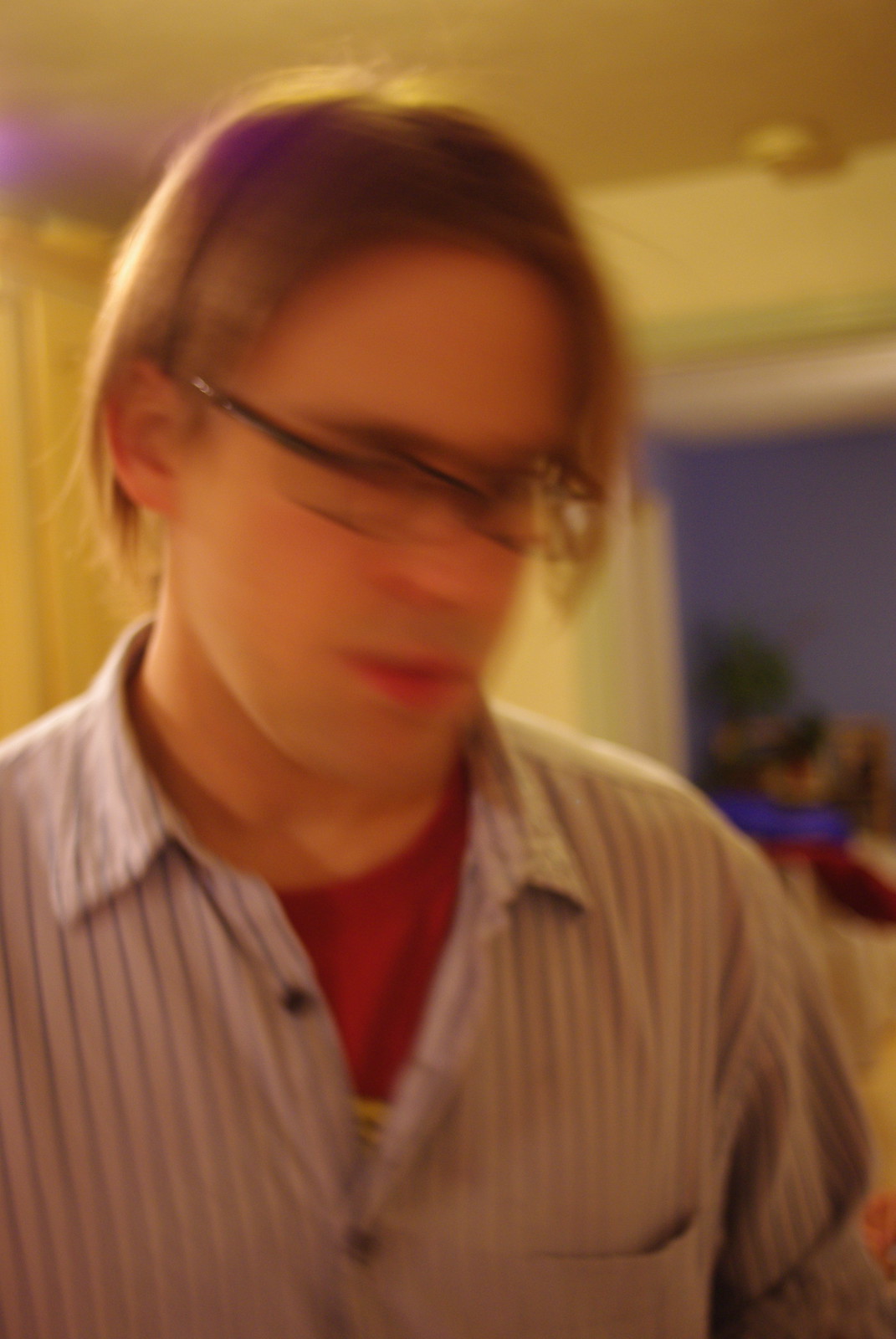In this blurry, somewhat out-of-focus photograph, there is a person whose age appears to be in the late 20s to late 30s, captured in portrait mode. The individual sports ear-length hair, parted on the left, and swept to the side, giving a slightly messy look. They are wearing thin black-framed glasses and facing downward toward the bottom right of the image. Their attire includes a mixed-pattern blue and white striped button-up shirt over a red t-shirt, which displays a hint of a yellow graphic logo. The background showcases an eclectic mix of colors and elements: the upper sections of the image reveal a yellow ceiling and walls, while the lower portion of the background through an opening or window has a light green wooden trim with a very light greenish-yellow paint. Beyond this opening is a darker blue area, possibly suggesting another room or a wall painted dark blue, with hints that could be indicative of an outdoor scene, maybe even a bright blue water source or sky. The combination of the light, movement, and moment at which the photo was taken results in a blurry image that captures the scene and subject dynamically but imprecisely.